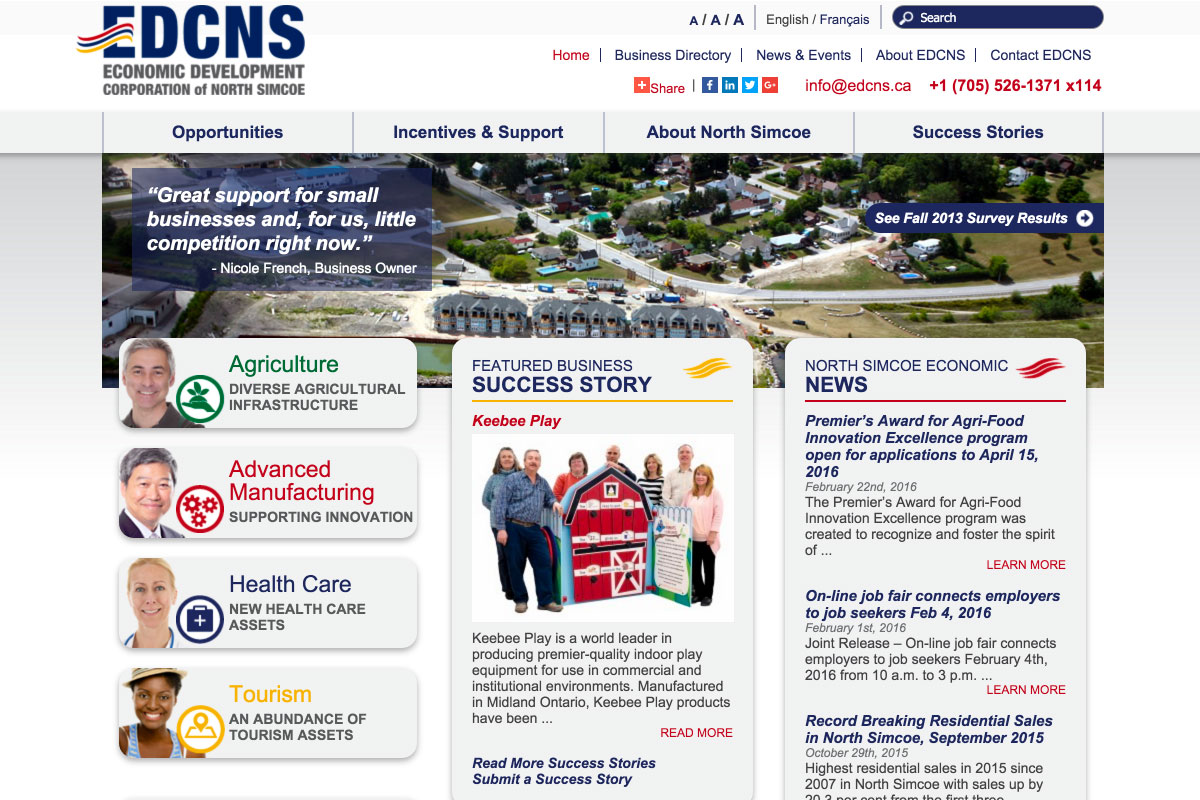This is a detailed screenshot of a web page belonging to the Economic Development Corporation of North Simcoe (EDCNS). At the top left corner, the EDCNS logo is displayed in dark blue lettering. On the right-hand side, a navigation menu includes tabs for "Home," "Business Directory," "News," "Events," "About EDCNS," and "Contact EDCNS," along with a phone number: 705-526-1371, extension 114.

Just below, four prominent tabs with a blue font on a gray background read: "Opportunities," "Incentives and Support," "About North Simcoe," and "Success Stories." An overhead aerial photograph of a town, showcasing roadways and houses, forms the backdrop. Overlaying this image are the words, "Great support for small businesses and for us, little competition right now," followed by a dash and the attribution, "Nicole, French business owner."

On the right side, there is a blue banner displaying "CFAW 2013 survey results." Beneath this, four rectangular boxes feature images of different individuals, each associated with a specific sector:
1. A white man with gray hair is labeled under "Agriculture."
2. An Asian man with black and gray salt-and-pepper hair, appearing to be in his 50s or 60s, is labeled under "Advanced Manufacturing" in red letters.
3. A white blonde woman with her hair pulled back, wearing a white blouse and a stethoscope around her neck, is labeled under "Healthcare."
4. An African-American woman with short hair and beautiful brown skin, wearing a tan hat, is labeled under "Tourism."